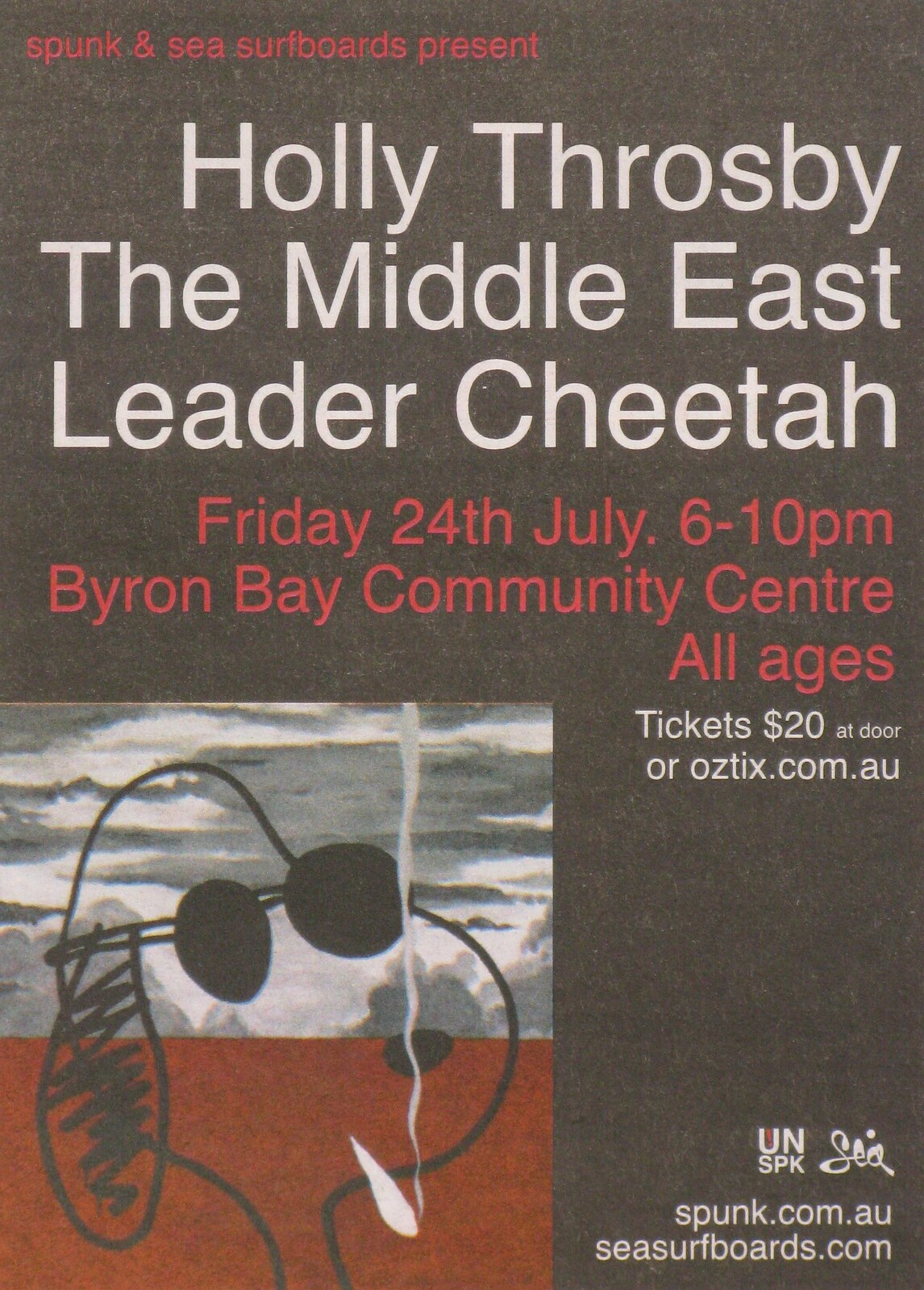The front page of the magazine has a predominantly gray backdrop with a mixture of red and white text, creating a striking visual contrast. Dominating the cover is a single, stylized image of Snoopy positioned at the bottom left. Snoopy is depicted smoking what appears to be a joint and is wearing dark sunglasses, adding to his "Joe Cool" persona. Below Snoopy, there are wispy, cloud-like formations in red and gray, giving a layered effect to the image.

From the top in bold red letters, it declares, "Spunk and C Surfboards Presents." Following below in white text are the featured artists: "Holly Throsby, the Middle East, and Leader Cheetah." Returning to red text, the details of the event are specified: "Friday, 24th July, 6 PM to 10 PM, Byron Bay Community Center, All Ages." Information about ticket availability follows, indicating that tickets are priced at $20 at the door or can be purchased online at ozticks.com.au. At the bottom, logos and additional URLs are presented, including "spunk.com.au" and "seasurfboards.com," along with UN, SPK, and SIA icons.

Overall, the magazine cover effectively combines a unique graphic with detailed event information, using a cohesive blend of gray, red, and white elements.